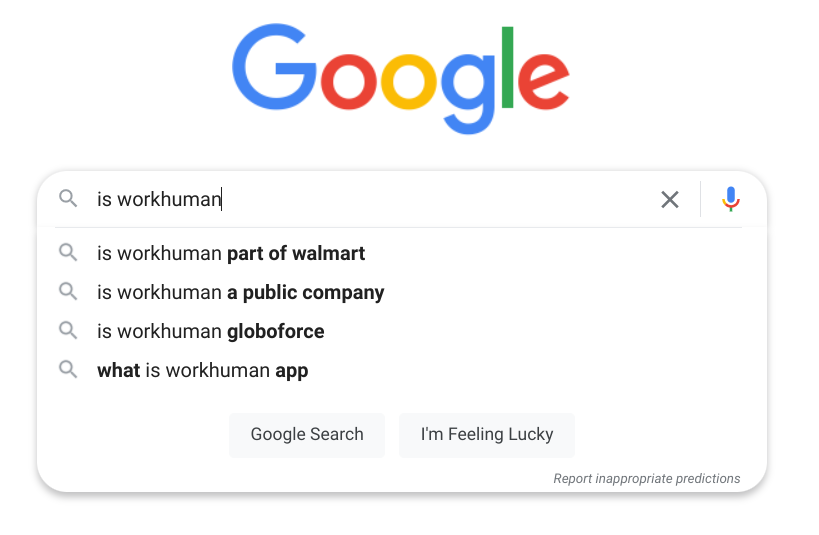The screenshot captures a Google search page. The iconic Google logo, with its blue, red, yellow, and green lettering, is prominently displayed at the top. Below it, the search bar features a magnifying glass icon on the left, followed by the text entry "is workhuman" (with no space between "work" and "human"). At the right end of the search bar, there's an "X" button for clearing the text and a colorful microphone icon that allows for voice searches, separated by a small vertical line.

The cursor is actively blinking at the end of the typed text. Underneath the search bar, Google provides several autocomplete suggestions, each beginning with a variation of the input text:

1. **is good work human part of Walmart** (with "part of Walmart" in bold to indicate the specific suggestion).
2. **a public company**.
3. **is global force**.
4. **what is workhuman app**.

These suggestions are likely based on popular searches related to the typed query.